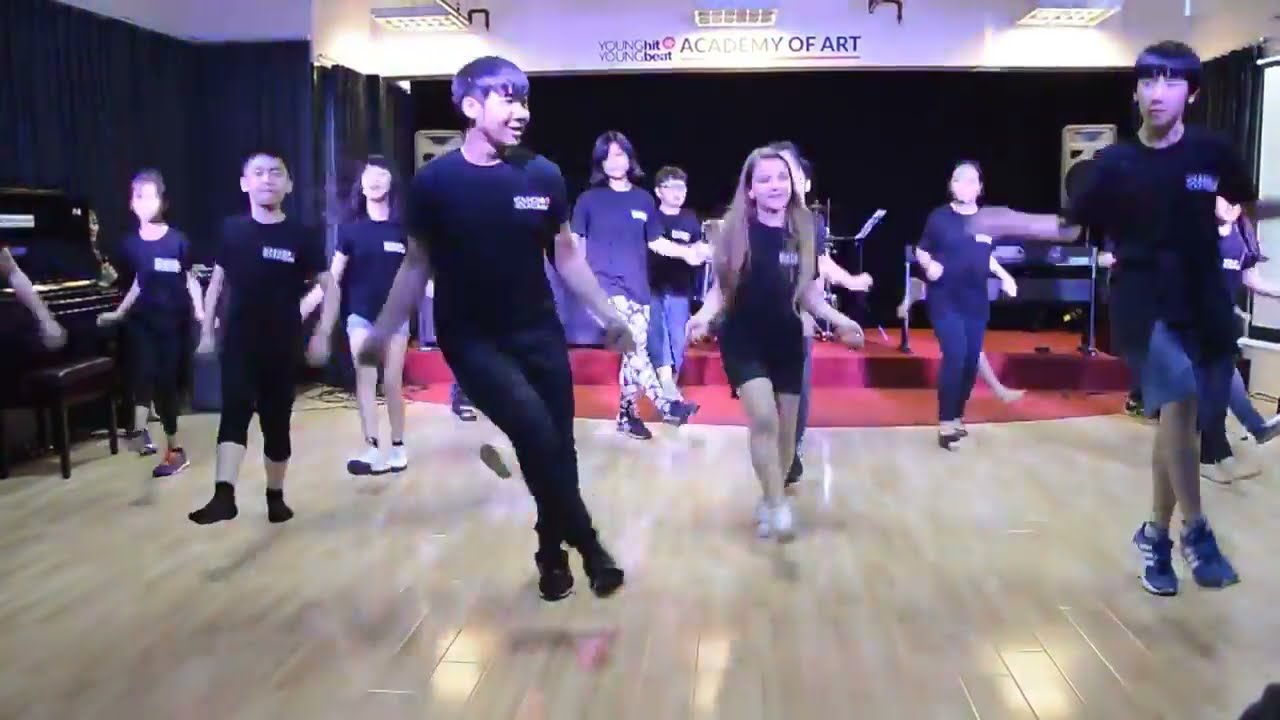The image depicts a lively scene of a youth dance class at the Young Hit, Young Beat Academy of Art, as indicated by a prominent sign in the background. The participants, primarily of Asian descent, are energetically dancing and leaping in a well-lit studio with a hardwood floor. They are mostly clad in black shirts emblazoned with the academy’s logo, and their attire varies from black pants and socks to denim shorts and tennis shoes. The dancers, likely teenagers, are a mix of boys and girls, all captured mid-motion with hands raised and feet stirring, suggesting a dynamic practice session. Surrounding them are black curtains and possibly a stage area with a drum set, hinting they might be rehearsing for an upcoming performance. The overall ambiance is one of enthusiastic rehearsal and dedication.